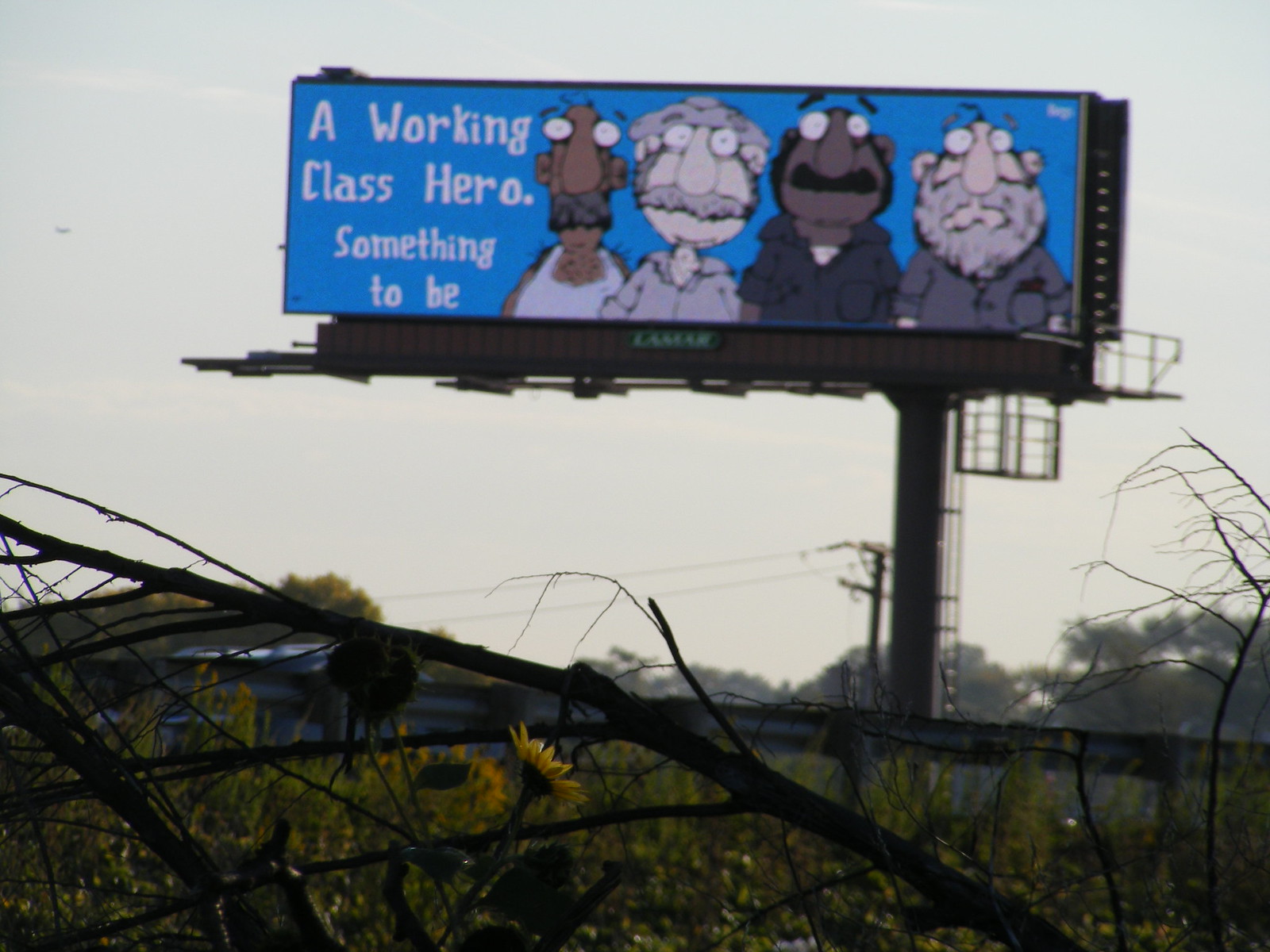In this striking photograph, a lone billboard stands out against a dramatically overcast white sky, lending an almost monochromatic backdrop to the vivid focal point of the image. Positioned within an overgrown, grassy meadow punctuated by downed tree trunks, the image is captured with a low perspective close to the ground, emphasizing the juxtaposition between the natural chaos below and the structured advertisement above. 

Dominating the right side of the scene is a major support beam, rising robustly from the earth to anchor the centrally located billboard. The billboard itself is set against a vivid blue background that starkly contrasts with the more muted tones of the scene. On the right-hand side of the billboard, a series of four cartoon-like characters draws immediate attention with their exaggerated features and bulging eyes. Representing a diverse array of ethnicities and appearing to be somewhat older, each character sports a distinctive mustache, adding a touch of whimsy to their stern visages.

To the left of these figures, white lettering boldly declares, "A working class hero, something to be," suggesting a broader societal message embedded within the playful art. This surreal blend of overcast nature and vibrant, eye-catching advertising creates a compelling tableau that invites deeper reflection.